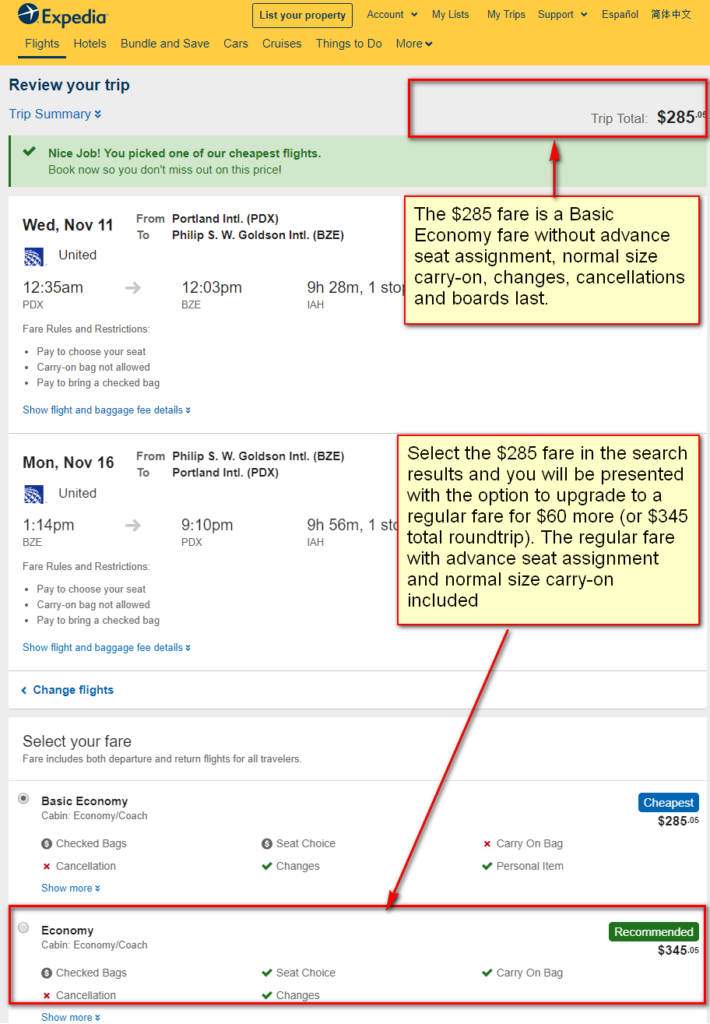In this detailed screenshot of the Expedia platform web page, we first notice the title bar at the top, which spans the entire width of the screen and is highlighted in a yellow rectangle. The upper left corner of this bar prominently features the Expedia logo, consisting of a white airplane inside a circle, accompanied by the word "Expedia" in bold black text with a capital "E". 

To the right of the logo are several menu buttons: the "List Your Property" button encased in its own rectangle, followed by "Account Menu," "My Lists," "My Tags," "Support," "Español," and an option with Chinese characters.

Below this primary title bar is the navigation menu for the webpage, offering different travel-related categories: "Flights," "Hotels," "Bundle and Save," "Cars," "Cruises," "Things to Do," and a "More" option.

Further down the page, there is a section titled "Review Your Trip" on the left, alongside a red box on the right indicating the "Total Trip Price." Within this red box, detailed fare information reveals that the $285 fare is for a basic economy flight, which does not include advanced seat assignment, normal-size carry-on bags, changes, cancellations, and boards last. This information is presented in a yellow box with a red outline.

The screenshot displays the travel dates "Wednesday, November 11th" for departure and "Monday, November 16th" for the return. At the bottom of the image, there are different types of selectable fares listed.